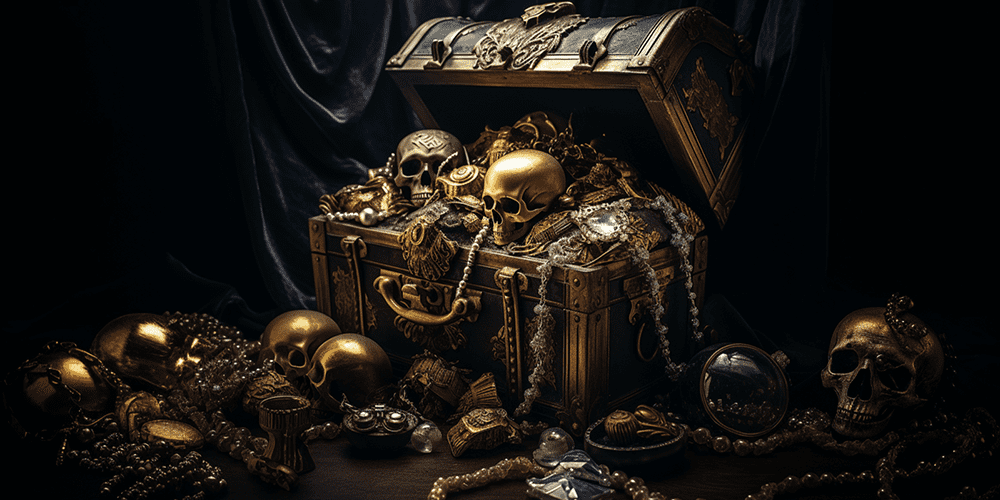The artwork depicts an ornate, black pirate's treasure chest with intricate gold accents, handles, and clasps, prominently placed at the center of the image. Its slightly open lid reveals a dazzling array of treasure, overflowing with gold and silver artifacts, jewelry, and multiple skulls, including a distinctive gold skull and a darker one with an etched symbol. The backdrop is dominated by a ruffled black curtain, adding a mysterious depth to the scene. Surrounding the treasure chest at the lower part of the image are scattered piles of treasure, including more skulls, cups, and strands of silver necklaces and pearls that have spilled out, creating a glittering foreground of gold and silver treasures against the dark, shadowy background.